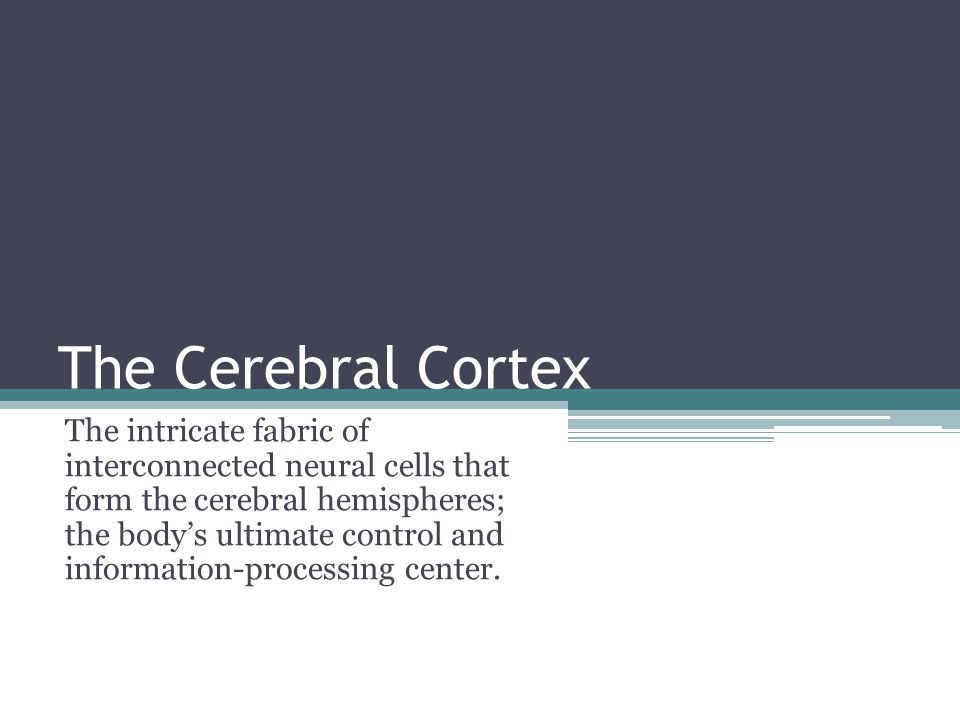This image resembles a slide from a PowerPoint presentation and is divided into two distinct halves. The upper half is a horizontal rectangle with a dark grey or black background and white text that reads "The Cerebral Cortex." Separating the two halves is a dark green slash blue line which transforms into a series of smaller lines, predominantly on the right side. The lower half has a white background with black text that reads, "The intricate fabric of interconnected neural cells that form the cerebral hemispheres; the body's ultimate control and information processing center." The visual is minimalistic, focusing on the stylistic use of colors and text, without additional graphics.